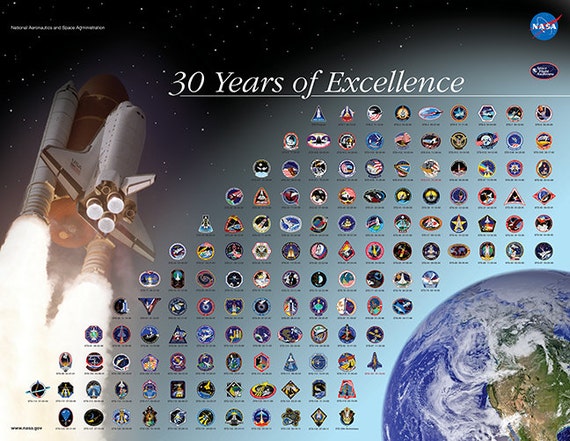This poster celebrates NASA's achievements with the theme "30 Years of Excellence." Prominently featured in the upper right corner, the NASA logo underscores the agency's significant milestone. Centered at the top, the phrase "30 Years of Excellence" is rendered in bold white text. The background showcases deep space, adorned with sparkling stars, creating a vast, celestial ambiance.

Dominating the left side of the image is a space shuttle, still equipped with its rocket boosters and external fuel tank, depicted in striking detail - the large orbiter is primarily white, with a central burnt-orange tank and white boosters releasing plumes of smoke. This illustrates a shuttle launch, emphasizing NASA's endeavors in space exploration.

In the lower right corner, a detailed photograph of Earth is visible. The image captures a segment of the Northern Hemisphere, highlighting North America amidst swirling white clouds over the blue expanse of the planet's surface.

Scattered across the middle portion of the poster are numerous patches, arranged in orderly rows. These patches, though hard to discern individually due to the image's resolution, represent various missions and accomplishments. They likely include numerous mission patches, which employees and astronauts would wear, signifying the many significant journeys undertaken over the years. This myriad of badges collectively narrates the rich history and numerous missions of NASA, encapsulating the agency's spirit and achievements in space exploration.